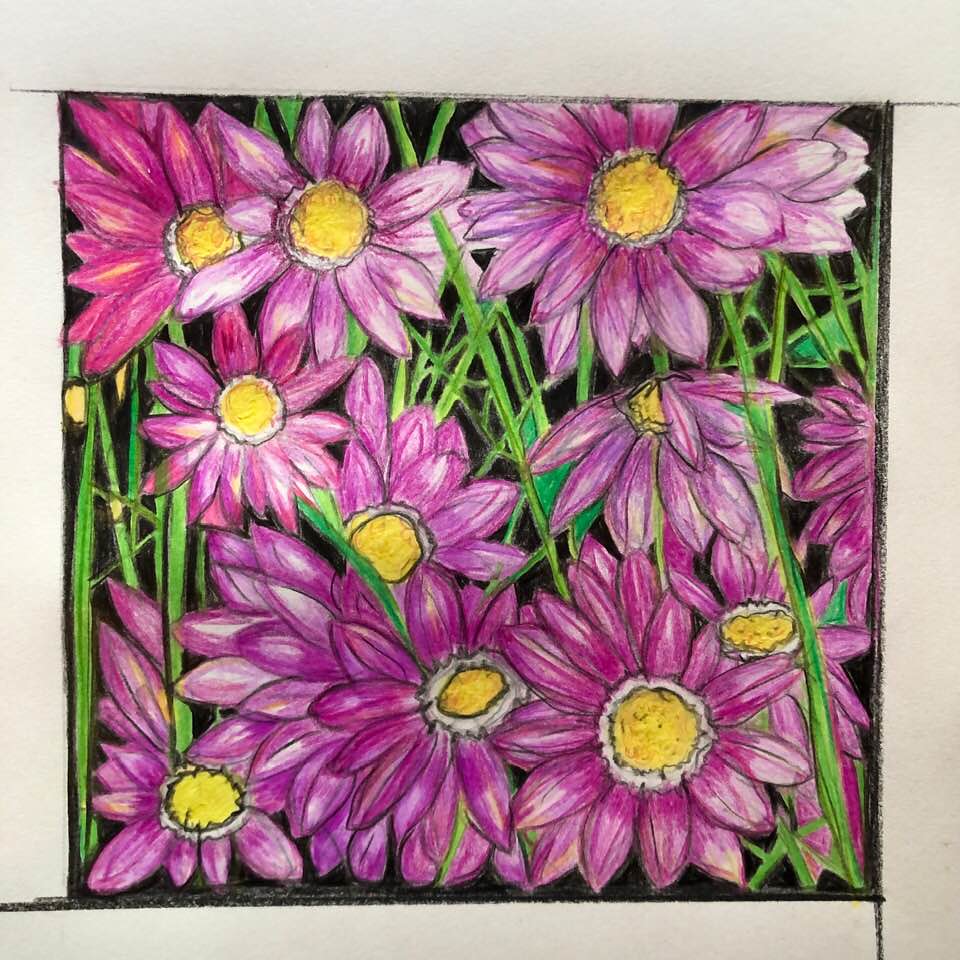This hand-drawn artwork showcases a vibrant collection of flowers against a stark black background, emphasizing the colorful hues. The flowers, numbering around 20, are depicted in a hodgepodge arrangement with overlapping petals in varying shades of magenta, pink, and purple. The centers of the flowers uniformly feature a white imperfect circle encasing a yellow imperfect circle, providing a striking contrast. The detailed rendering—potentially created with colored pencils or charcoal—reveals individual lines and various coloring intensities within the petals. Green stems interweave behind and in front of the flowers, accompanied by a few green leaves, all contributing to the complex composition. The entire image is bordered by a hand-drawn black frame, which adds to the artistic, almost whimsical, feel of the piece. The black background, though not a natural setting, effectively highlights the vivid colors of the flowers.